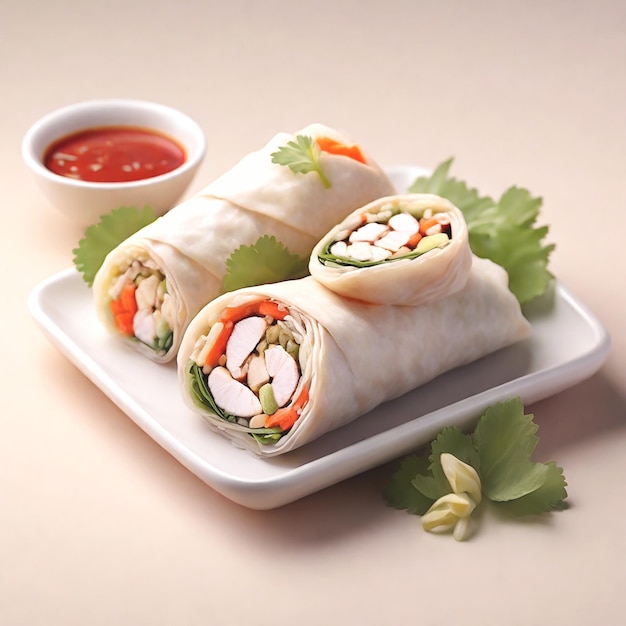In this vivid close-up photograph of food, two veggie wraps are elegantly presented on a square white plate, placed over a pinkish cream background. The wraps, made with an off-white, flower-like tortilla, are cut down the center, displaying a colorful assortment of ingredients including orange carrots, various beans, leafy greens, potential mushrooms, and white seed-like elements. Both wraps sit side-by-side, with a small cutout portion of one wrap thoughtfully placed on top of the right wrap. The plate is adorned with decorative green leaves arranged strategically—between the wraps, atop the left wrap, and around the plate's borders, with one leaf extending off the plate on the bottom right. Additionally, a small bowl brimful with red dipping sauce, speckled with seeds, is positioned at the top left corner of the plate, contributing to the dish's vibrant and fresh presentation.